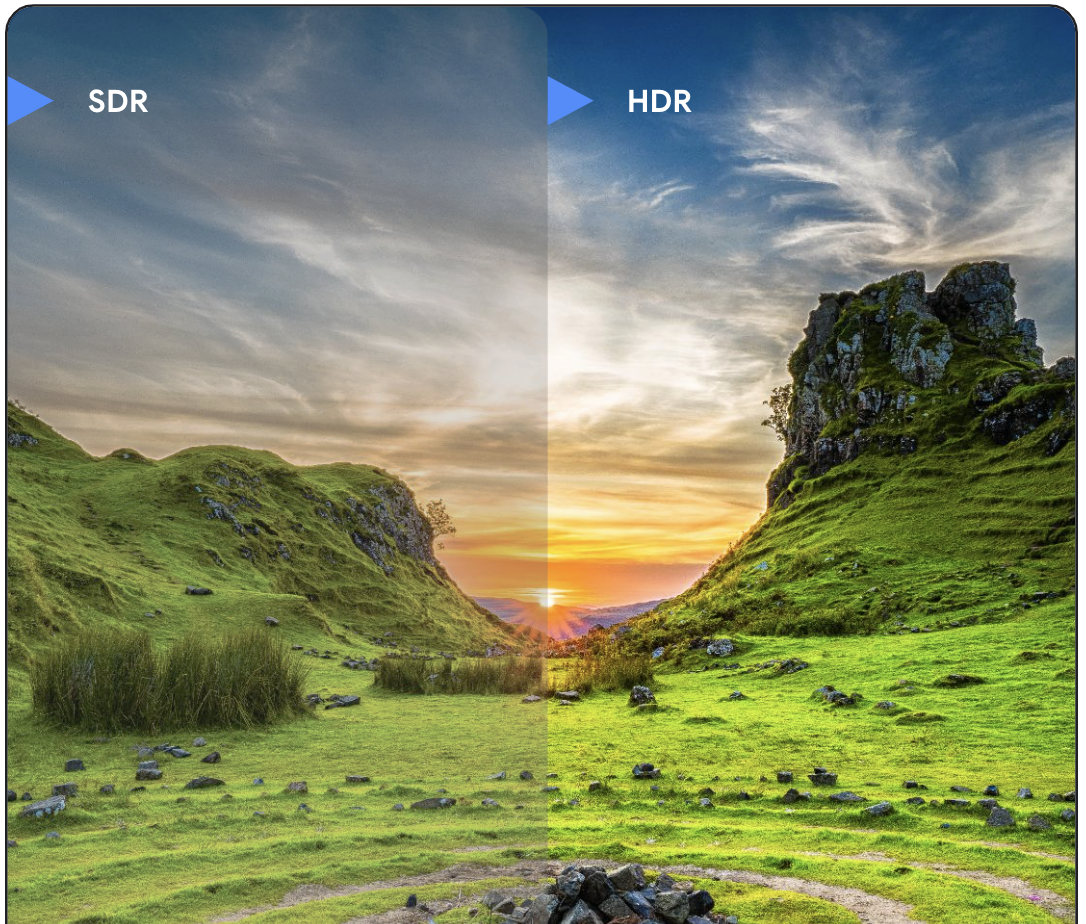The image is a side-by-side comparison clearly divided into two sections: SDR on the left and HDR on the right. Each section is labeled at the top left corner with a blue play symbol—SDR in white text on the left and HDR on the right. The photo captures an open field adorned with vibrant tall grasses, flanked by majestic cliffs. The landscape features a striking valley, and in the distance, the sun is either rising or setting, casting a beautiful array of colors across the sky. The SDR side appears dull and muted with low contrast, exhibiting a grayish tone and less defined details. In contrast, the HDR side is vivid and crisp; the colors—ranging from deep oranges and yellows to rich blues—are exceptionally radiant, bringing the scene to life. This stark comparison emphasizes the enhanced clarity and color depth of the HDR side, highlighting every detail from the moss-covered cliffs to the wispy clouds in the colorful sky.